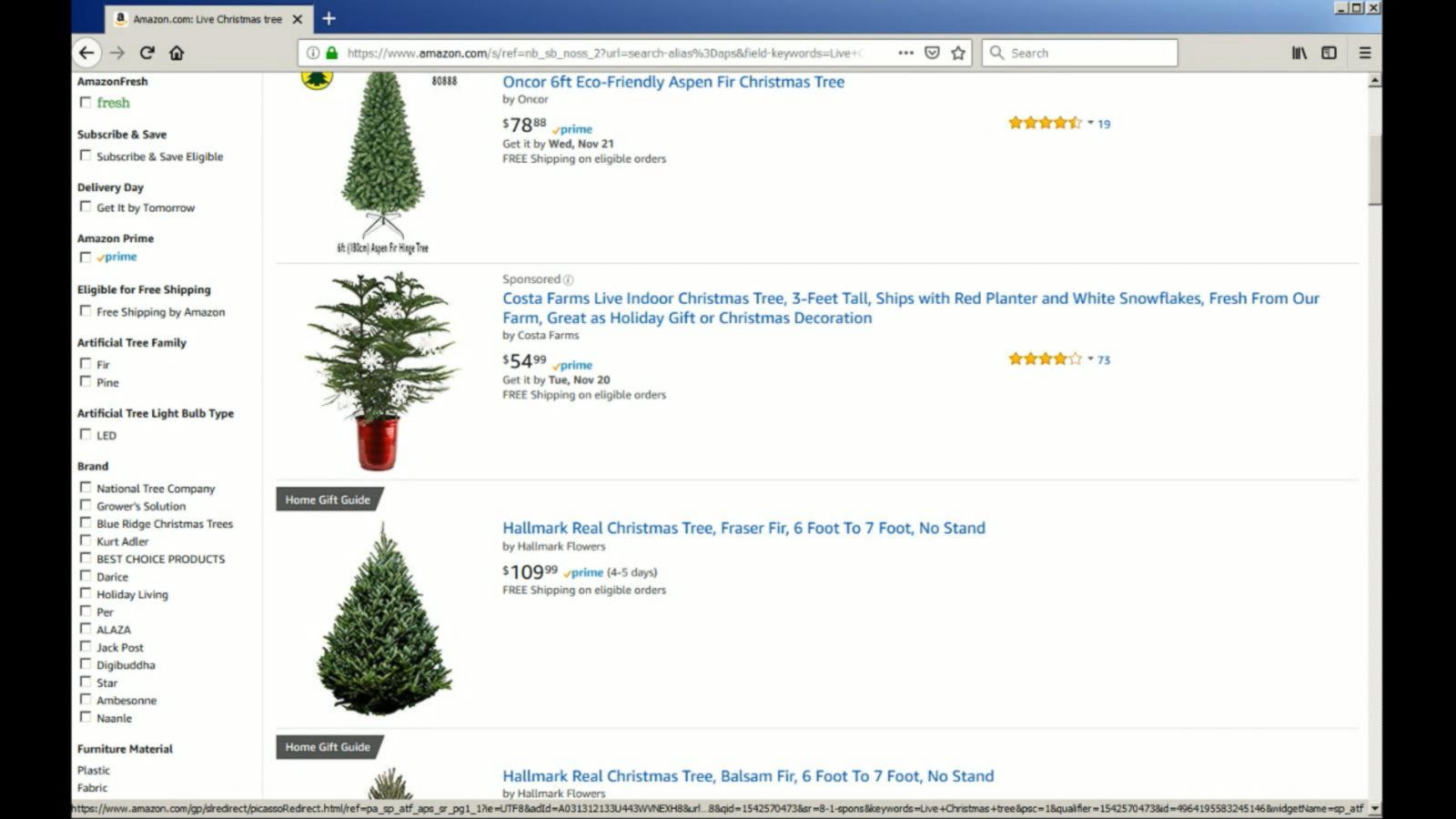The image depicts a computer browser window displaying a webpage on Amazon.com focused on live Christmas trees. The orientation of the image is a rectangle with the longer sides extending horizontally, bordered by thick black lines on the left and right.

At the top of the browser, the background is gray, and it shows a single open tab labeled "Amazon.com, live Christmas tree." Below the tab, there is a row of navigation icons including a left arrow, right arrow, refresh icon, home icon, and a star for bookmarking. Adjacent to these icons is an empty search box with a search icon and the word "search" inside it. Additional utility icons are located on the far right.

The main section of the webpage is divided into two primary columns. The left column features various filters and categories for selecting a Christmas tree. These options include "Subscribe and Save," "Amazon Fresh," "Delivery by," "Amazon Prime," and "Eligible for Free Shipping." There are also detailed categories such as "Artificial Tree Family," "Artificial Tree Light Bulb Type," "Brand," and an extensive list of brands. Further down, there is a filter for "Furniture Material."

The right column prominently displays three images of different Christmas trees. Each image is accompanied by detailed labels, names, and prices, providing various options for customers to compare and choose from.